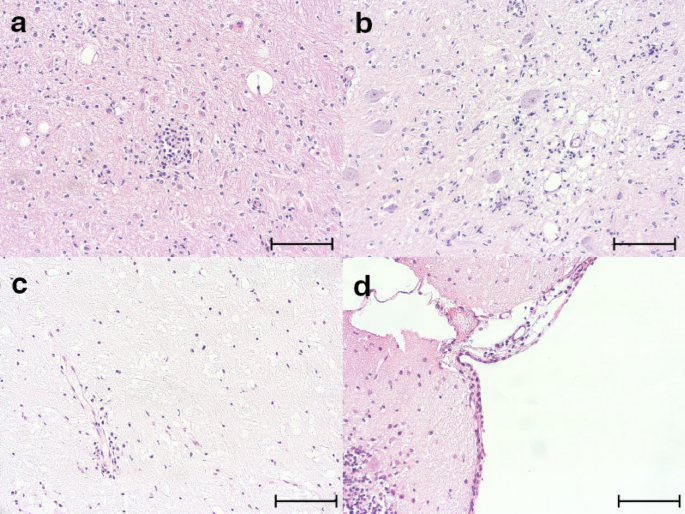The image is divided into four equal, square frames labeled A, B, C, and D, arranged in a larger rectangular or square formation with A and B on top and C and D on the bottom. Each frame showcases a microscopic view of some kind of cells or tissue, resembling an abstract painting. Frame A features a predominantly pink background with white striations and purple spots, as well as some translucent oval or spherical white objects. There's also a black measuring bar at the bottom of the frame. Frame B is nearly identical to A, sharing the pink background, purple spots, and black measuring bar. Frame C has a lighter pink background with fewer purple spots, and Frame D is characterized by more white areas than pink, with deep purple and pink spots scattered throughout. The overall aesthetic of the images is visually appealing, with vibrant pinks, purples, and whites making the microscopic details look almost like a delicious ice cream treat.